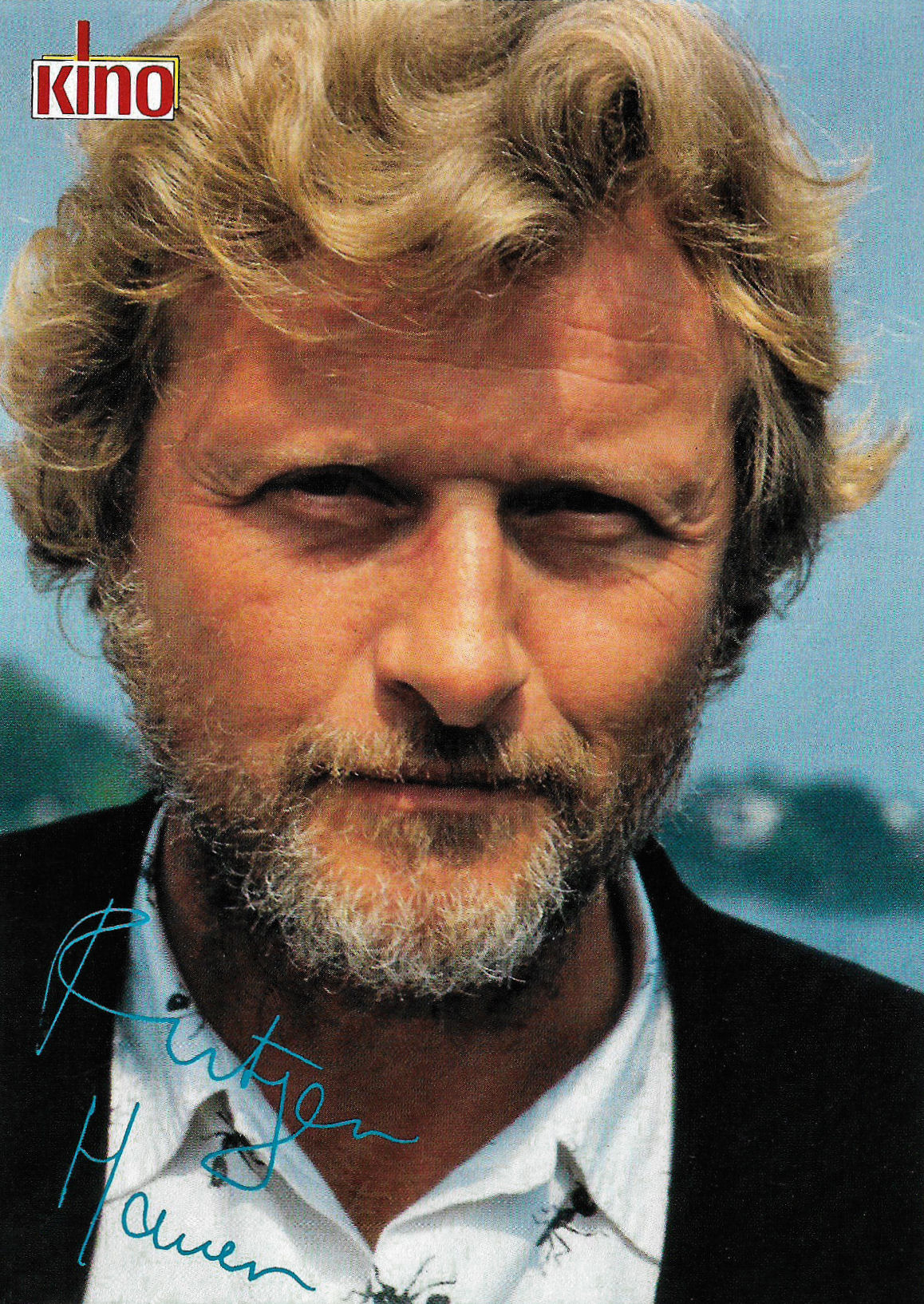The photograph features Rutger Hauer, known for his iconic role as Roy Batty in "Blade Runner." Captured in his middle-aged years, Hauer sports short, curly blonde hair and an unshaved beard predominantly blonde with speckles of gray, particularly on the chin. He is dressed in a stylish black suit paired with a unique white shirt adorned with illustrated ants. The backdrop showcases a blurred seaside landscape, featuring blue skies, water, and indistinct mountains, adding a serene ambiance to the image. In the top left corner, there is a logo reading "Kino," and at the bottom left, Hauer's autograph is prominently displayed in light blue lettering. The photograph has a somewhat vintage quality, suggesting it may have been printed on older paper, contributing to its nostalgic aesthetic.